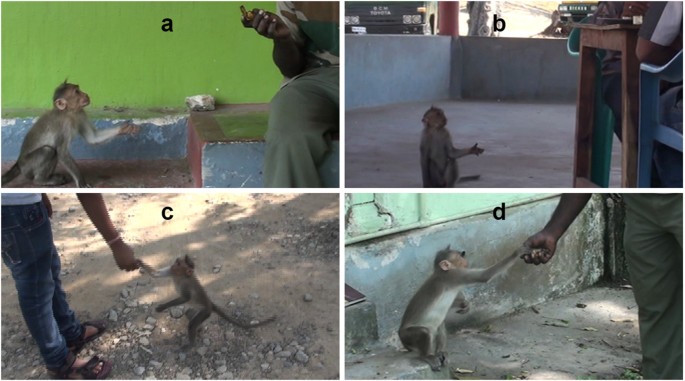The image comprises four amateurish, tourist-like photographs, each labeled A, B, C, and D, depicting a small spider monkey interacting with humans and its environment. In each photo, colors range from green, black, white, blue, brown, tan, teal, gray, and a hint of orange in the top right image. 

In the top left photo (A), the monkey is positioned against a green background with a cement floor. A man is visible sitting on a bench on the right side, likely offering something to the monkey, which has its hand raised. 

In the top right photo (B), the monkey is situated in a different setting with a cement floor and a small wall, which might be part of a truck park. The monkey appears to be looking up at people seated at a nearby table.

The bottom left photo (C) shows the monkey on a rocky, dirt ground. Here, a man is bending down with just his lower body visible – legs, shirt, and flip-flops – as he shakes the monkey's hand or possibly offers him food.

In the bottom right photo (D), the scene shifts to a blue background. The monkey is seated, reaching out to shake or take something from a man's outstretched hand.

Overall, the photos capture the monkey performing various interactions, primarily with human hands, in diverse environments.